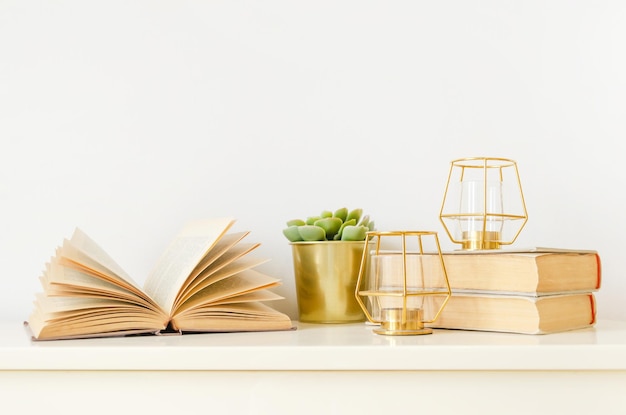This is a color photograph showcasing a minimalist, white table set against a plain, solid white background. On the left side of the table, an open book with pages seemingly ruffled by an invisible breeze, stands out with its yellowy-green colored pages. Adjacent to the book sits a gold-colored, cylindrical planter housing a light green succulent. Further to the right, a stack of two closed books is positioned, revealing only their pages and not their spines. On and in front of this stack are two identical candle holders with hexagonal or cubical glass frames and brass linings, containing gold tea lights, adding a subtle touch of elegance to the otherwise austere setup.